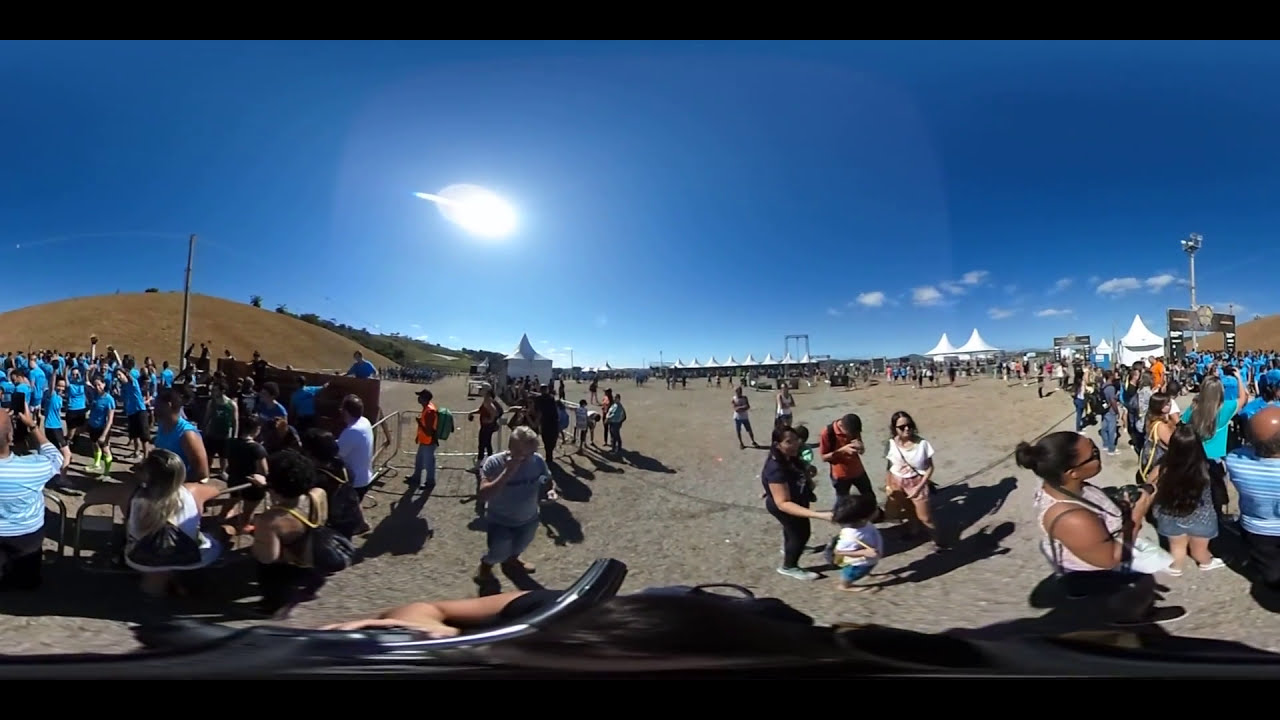A bustling, sunlit festival scene unfolds in an open field, thick with summer crowds dressed in shorts and short-sleeved shirts. A striking blue sky dominates the top half of the image, with a bright beam of sunlight piercing through white clouds on the upper left, contrasting with the clearer right side. The panoramic view captures a sandy, grey terrain scattered with mounds of brown dirt and patches of grass. To the left, an electric pole rises above the scene, while in the distant background, cone-shaped white tents or gazebos pepper the landscape.

A noteworthy gathering of individuals stands out in matching sky blue T-shirts and black pants, hinting at a possible group affiliation. These figures are concentrated more towards the left side of the image, where most are standing, with some sitting in front. Mixed casually among them are people of various ages, from children to teenagers, dressed in varied clothing.

In the foreground, part of the dark-haired photographer is visible, their hand gripping the camera. Despite the lack of a clear thematic element, the image vividly depicts a well-attended, outdoor festival atmosphere with numerous participants and diverse activities unfolding against the vibrant backdrop of a summer sky.